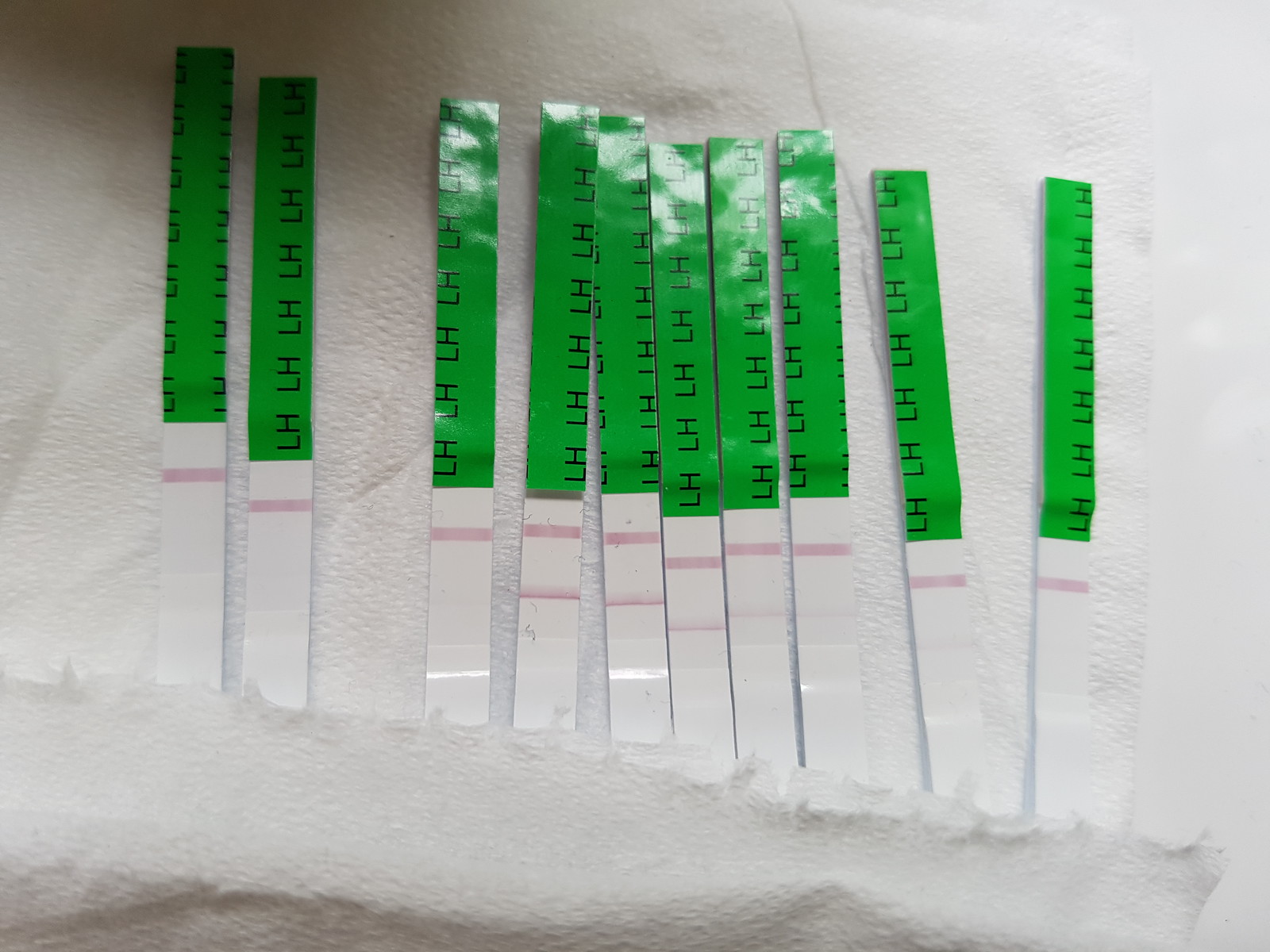A detailed photograph showcases a collection of ten ovulation test strips arranged on a white paper towel. These strips are predominantly green at the top, emblazoned with the repeating capital letters "LH," and transition to white at the base, where various bars and codes are visible. The strips are methodically laid out: two strips are placed on the left, six are clustered together in the center, and another two are positioned on the right. The clear delineation of colors and markings on the strips indicates their specific purpose and ensures ease of identification and use.